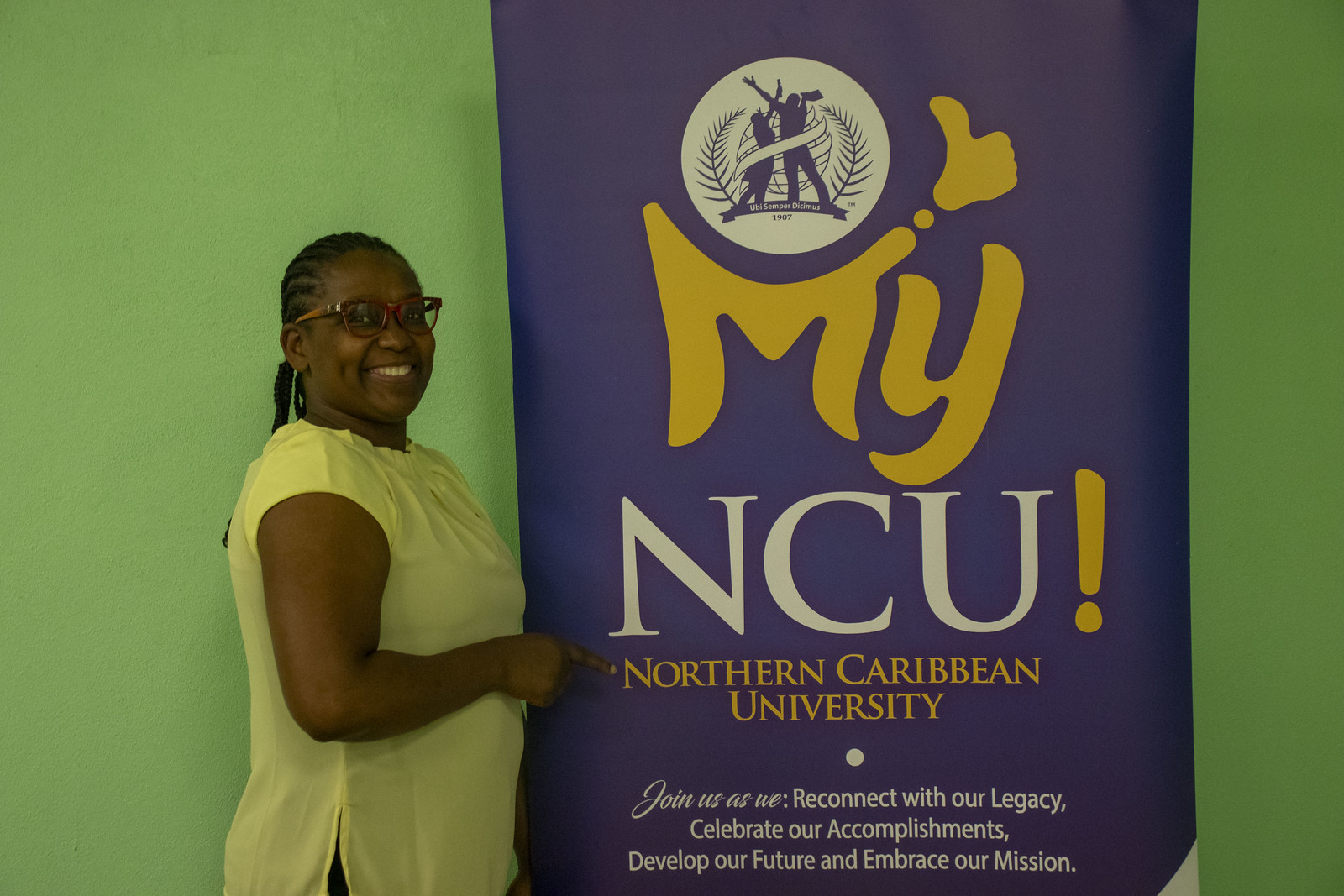At an outdoor event, a young African-American woman stands proudly beside a dark blue vinyl banner with white ornamental text that reads "MyNCU!" The "My" features a cleverly designed iconic thumbs up at the top of the "M." Below this, "NCU" is displayed in slightly sloped white text, accompanied by a smaller white asterisk. The full name "Northern Caribbean University" is written in bold white text, followed by an inspirational message in smaller print: "Join us as we reconnect with our legacy, celebrate our accomplishments, develop our future, and embrace our mission." Above the word "My" is the university's crest, depicting two silhouetted figures with arms raised towards the sky, standing against a globe, surrounded by laurels on either side, and the motto "Ubi Semper Dicamus 1907" inscribed below. The woman is dressed in a short-sleeved yellow blouse, her hair pulled back in braids, and she wears large red spectacles, beaming with a bright smile as she poses.